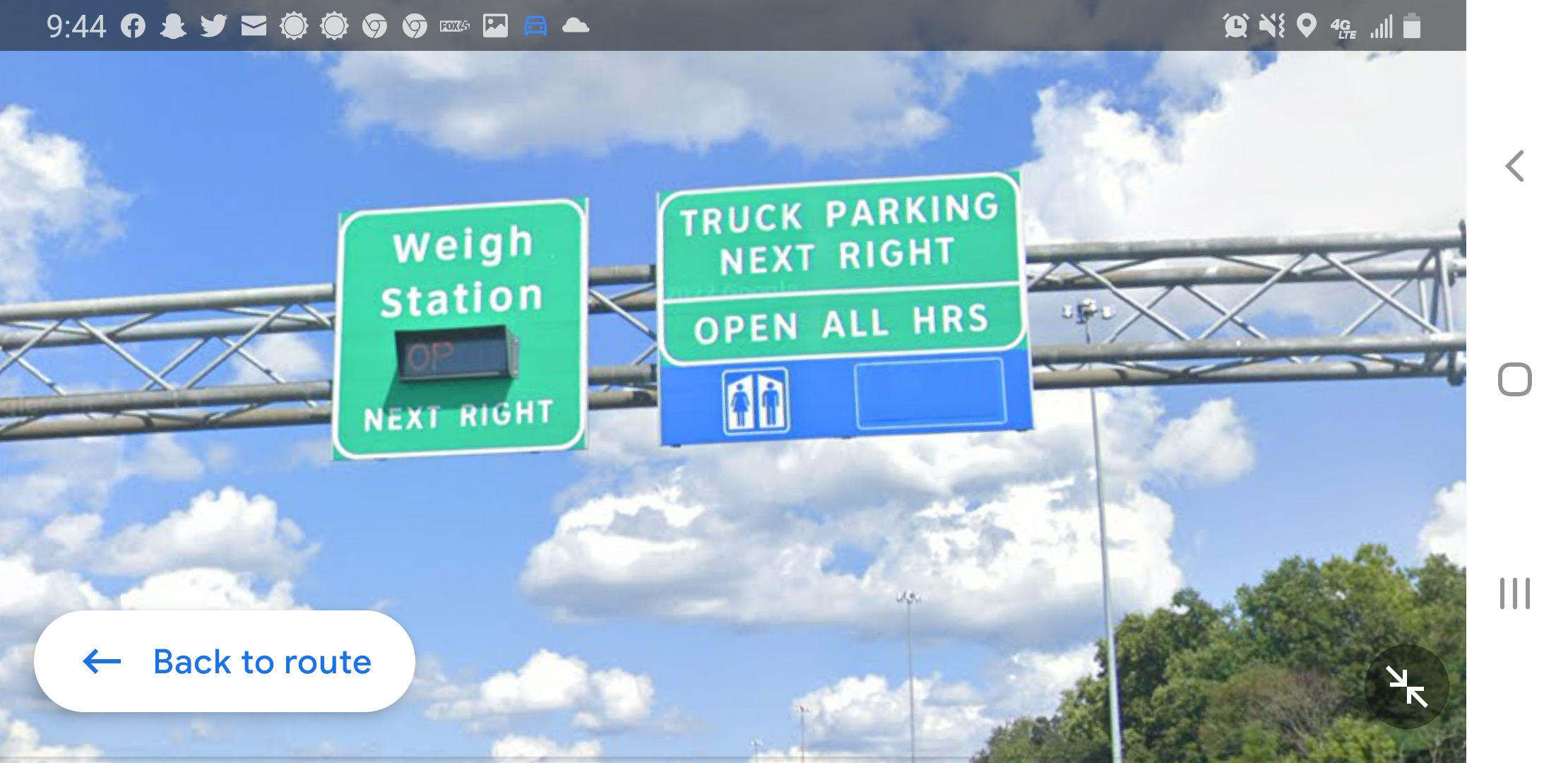Screenshot of a driving GPS interface. Across the top are various icons, including the time "9:44" and indicators for an alarm, 4G connectivity, battery life, and signal strength. The image prominently features the view of a highway, particularly the metal scaffolding that supports overhead road signage. On the left side of the display is a green rectangular sign with a white reflective border reading "Weigh Station Next Right." Adjacent to it is an electronic sign displaying "OP," and further to the right is another sign stating "Truck Parking Next Right, Open All Hours." Below these signs, there is a blue section with symbols indicating restrooms for men and women. In the lower left corner of the GPS interface, the phrase "Back to Route" can be seen, indicating a navigation option. The screenshot represents a digital depiction of a real-world highway scene and not an actual live view.